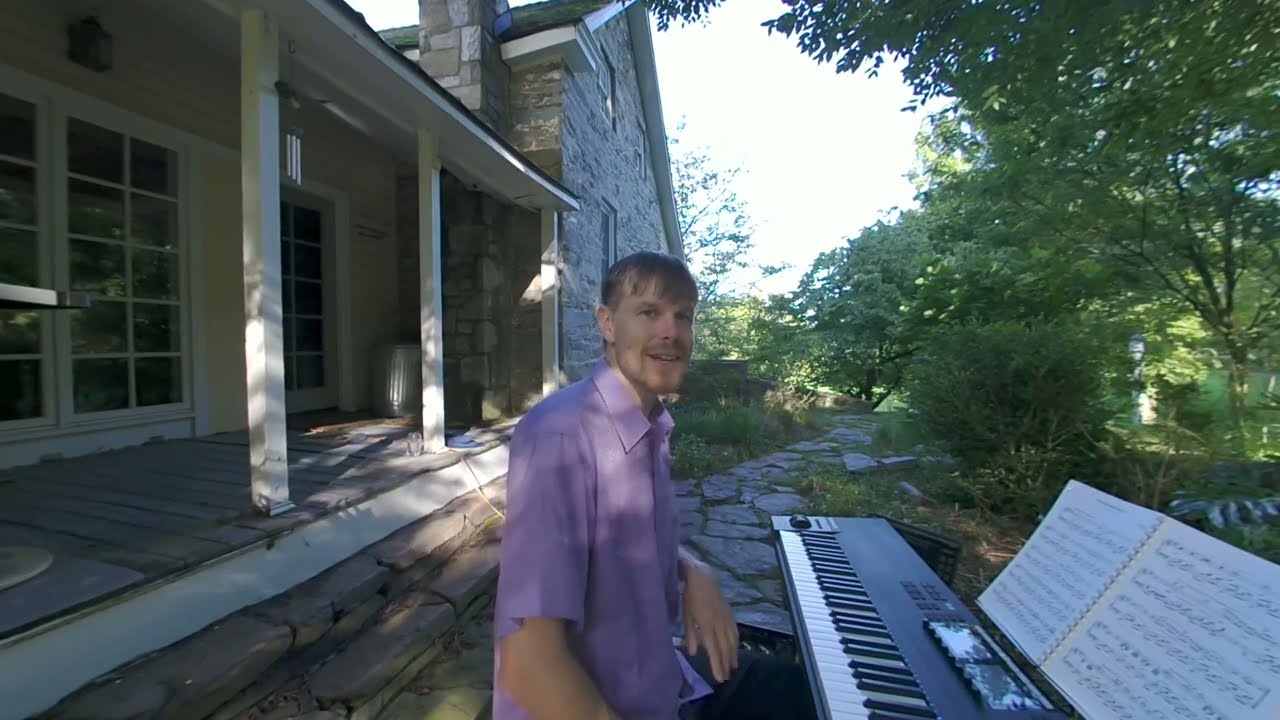In this vibrant summer photo, a young Caucasian man with short brown hair and a beard sits on a chair in a garden area just outside his home, ready to play his black and white electric keyboard. He is wearing a light purple shirt and is looking at the camera with a slight smile. The keyboard has an open music book on its stand, displaying sheet music for his upcoming performance. Surrounding him are verdant trees and bushes, and directly behind him is a picturesque stone and wood house. The house features large glass doors, white wooden support pillars for a long porch, and a stone chimney. A cobblestone walkway lies just behind where he sits, leading to the house. A trash can is tucked away in the corner of the porch. Sunlight illuminates the scene, enhancing the lush green hues of the garden and the bright sky visible through the trees. The overall ambiance suggests a serene, sunny summer day.